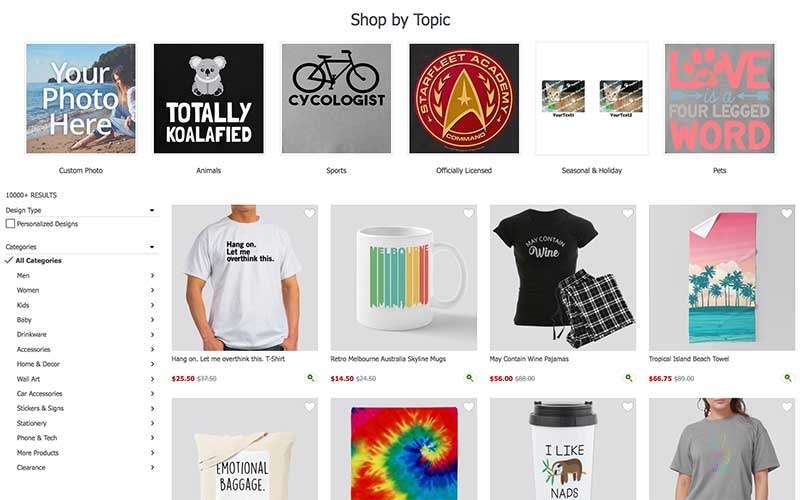On this vibrant and bustling shopping website, visitors are greeted with a colorful and dynamic interface dedicated to customizable printed merchandise. Dominating the top of the page is a prominent banner stating "Shop by Topic," followed by a horizontal row of six engaging, illustrative squares showcasing various design themes.

1. **Square 1:** Displays "Your Photo Here" for personalized items.
2. **Square 2:** Features an adorable koala captioned "Totally Koala-fied."
3. **Square 3:** Illustrates a bicycle with the quirky text "Psychologist" with a playful 'C.'
4. **Square 4:** Exhibits a red circle with "Star Fleet Academy."
5. **Square 5:** Shows two images of the same cat with unreadable text.
6. **Square 6:** Contains the phrase "Love is a Four-legged Word" in bold red letters.

Beneath these example squares, the topics are clearly labeled: Custom Photo, Animal, Sports, Officially Licensed, Seasonal & Holiday, and Pets. 

The main shopping area is a lively mix of products:

- A white t-shirt with the phrase "Hang on, let me overthink this."
- A rainbow-colored mug with "Melbourne" inscribed.
- A black t-shirt reading "May Contain Wine."
- A tropical-themed poster depicting palm trees and a sunset.
- A tote bag adorned with the phrase "Emotional Baggage."
- A square displaying a tie-dye pattern.
- A mug that humorously states "I like nads" with an image of an indeterminate animal.
- A plain gray t-shirt.

On the left side of the page, a navigational menu offers easy access to various product categories:

- Men
- Women
- Kids
- Baby
- Drinkware
- Accessories
- Home Decor
- Wall Art
- Car Accessories
- Stickers & Signs
- Stationery
- Phone & Tech
- More Products
- Clearance

This meticulously arranged interface not only highlights a wide array of customizable products but also ensures a user-friendly shopping experience.